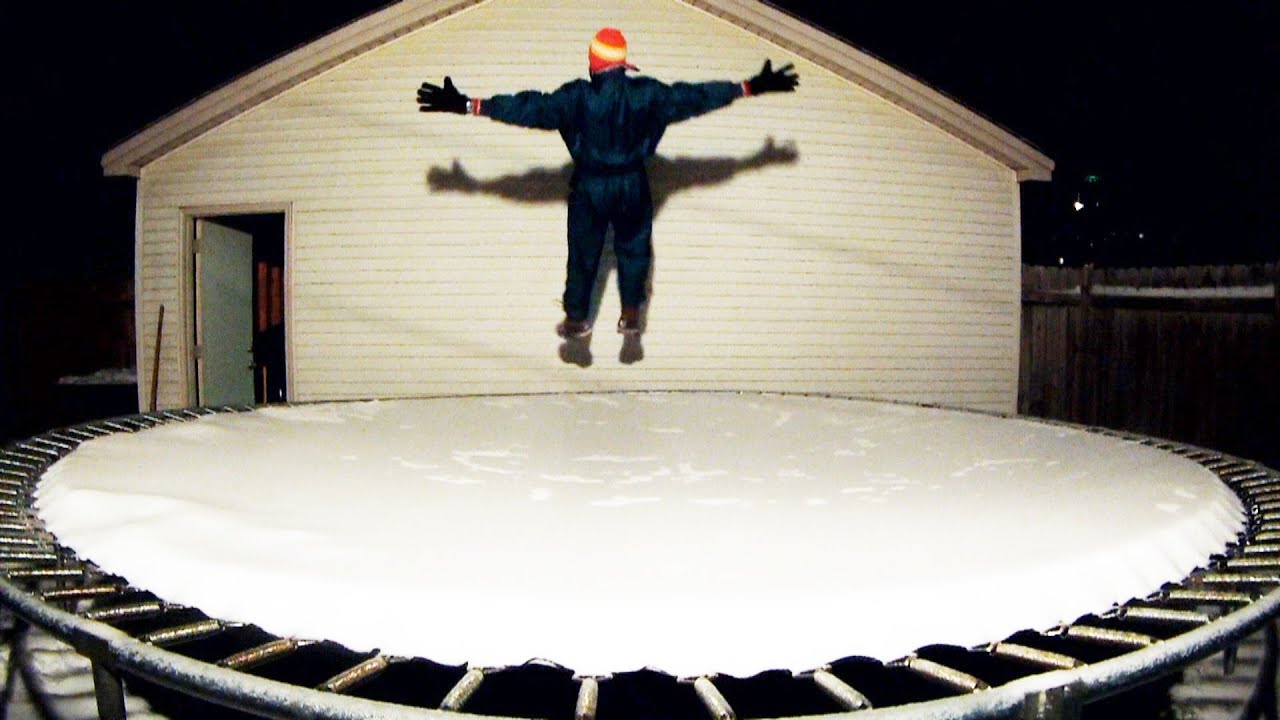The photograph captures a nighttime winter scene in a backyard or side yard, showcasing a snow-covered trampoline positioned against an old, rusty shed or garage with an open door on the left side. A thick layer of snow blankets the trampoline, revealing footprints where someone has recently climbed up. The focus is on a person dressed in a dark blue snowsuit and black gloves, wearing an orange beanie adorned with a yellow and white stripe. This individual is caught mid-jump, about two feet above the trampoline with arms extended outward. Their back is to the photographer, suggesting they may have leaped from the edge of the trampoline or a nearby structure. To the right of the shed is a wooden stockade fence, also dusted with snow, with the individual's shadow faintly cast on the shed wall by a light source. The overall scene is dark, adding a sense of stillness and mystery to the playful moment captured.